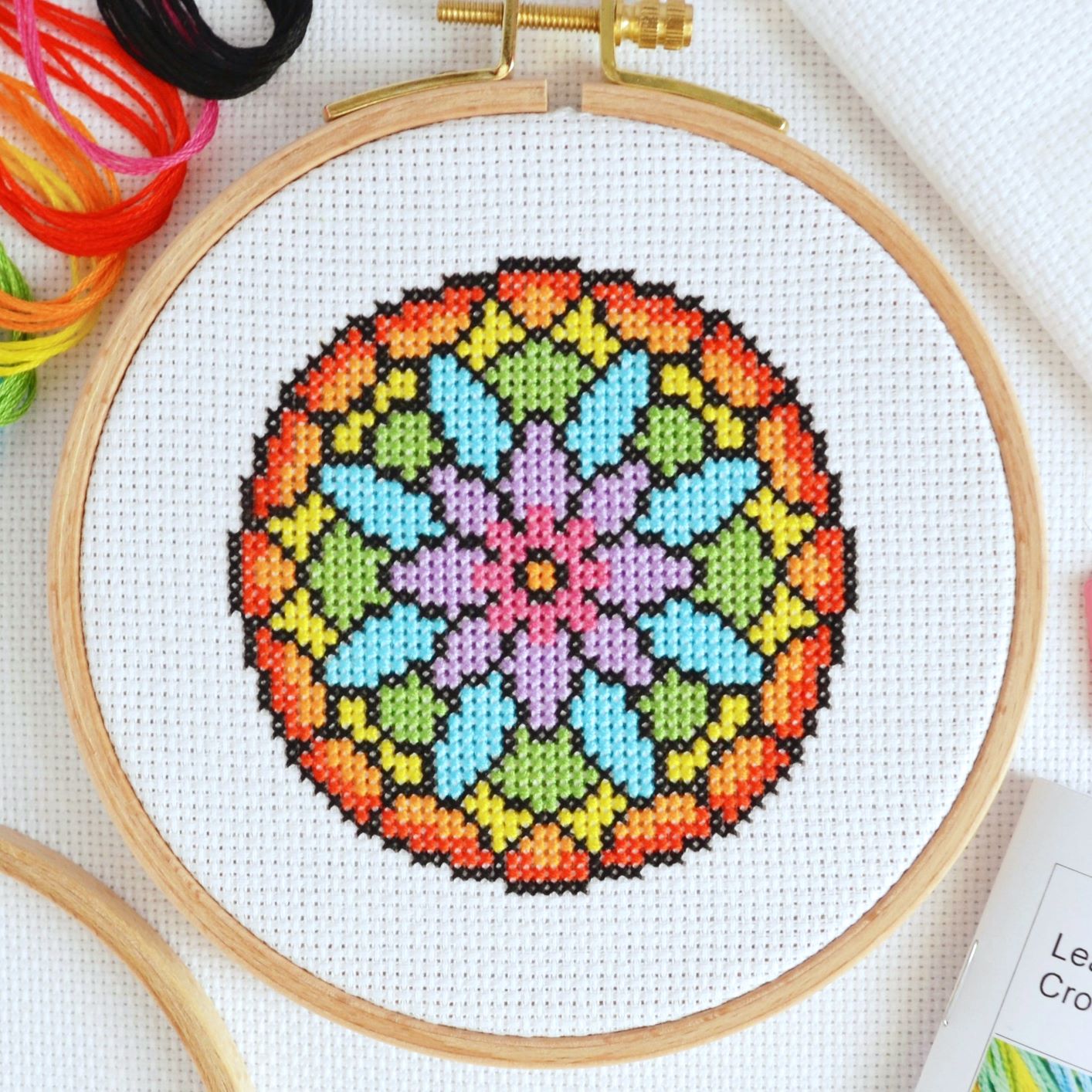The image captures a detailed close-up of a cross stitch project held within a circular wooden embroidery hoop, which has a golden tightener at the top. The fabric used for the cross stitch is white, featuring a meticulously crafted flower as the centerpiece. This flower begins with an orange center, extending outward with patterns of pink, purple, and blue stitching. Surrounding the flower are geometric designs in shades of green, yellow, orange, and red, all outlined in black, which also provides definition to the flower itself. Underneath the hoop, additional cross stitch fabric is visible, along with another embroidery hoop partially pictured in the bottom left corner. Scattered around are various colors of embroidery floss including green, yellow, orange, red, pink, and black, and a partially visible instruction manual located in the bottom right corner of the frame.